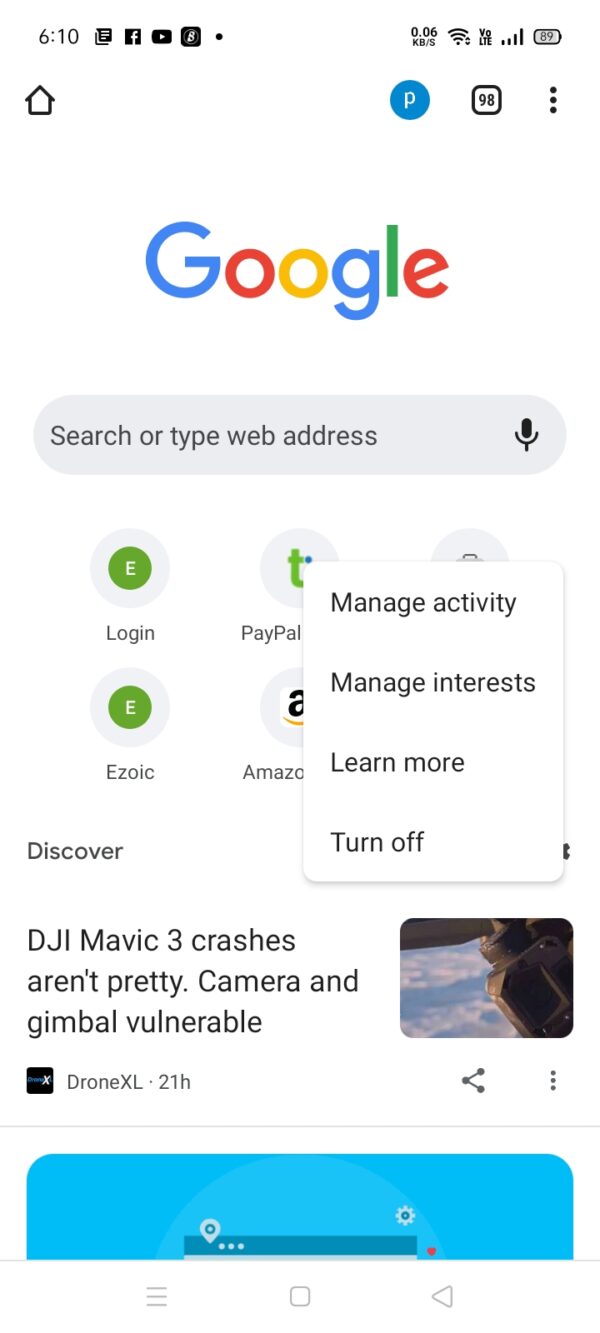The image depicts a smartphone screen open to a Google-branded website at 6:10 p.m. The top status bar of the phone displays various icons, including those for Facebook, YouTube, and some others, alongside signal bars, internet connectivity indicators, and additional icons. Below this, there's a navigation section featuring a home icon, a blue circle with a 'P', a black outlined box displaying '98', and an ellipsis icon (three dots).

The main content of the screen starts with the Google logo and a search bar. Beneath the search bar, there are six clickable icons, starting from the left: Log on, E-ZAC, PayPal, Amazon, with two other icons obstructed by an overlaying box labeled "Manage activities", "Manage interest", "Learn more", and "Turn off".

To the left of this section, the word "Discover" is displayed. Further down, the screen shows a headline that reads "DJI Mavic 3 crashes aren't pretty; camera and gimbal vulnerable", accompanied by an image of unclear detail. This article is credited to "Drone XL" and was published 21 hours ago. A blue box is below this line, but its contents are obscured.

At the very bottom of the screen, the standard navigation options are visible, including back and other common phone functionalities.